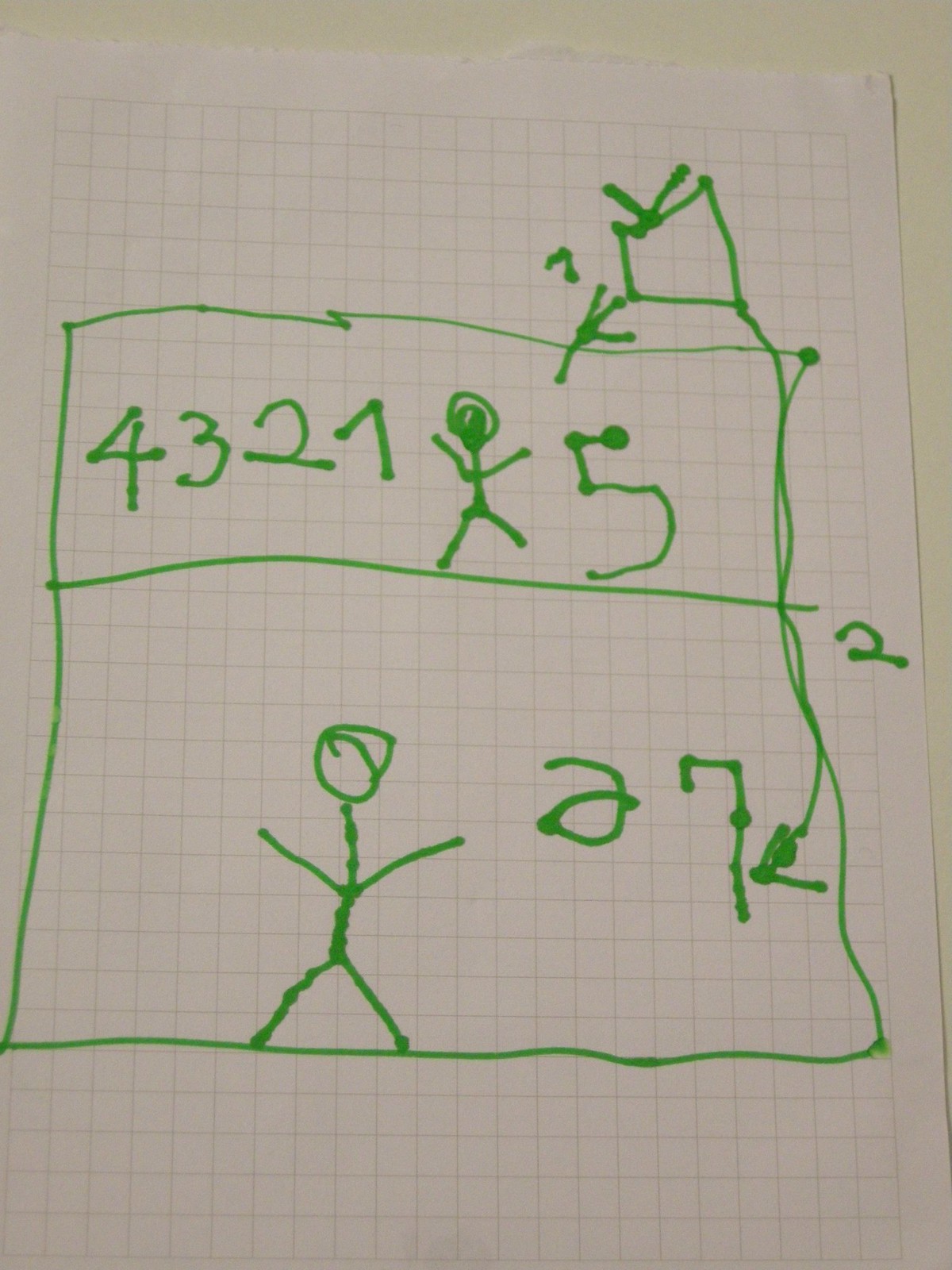The image showcases a structured grid composed primarily of squares. At the top of the grid, there is a small rectangle labeled "4, 3, 2, 1" beneath which a human figure with arms and legs outstretched is depicted. Directly below this is another label featuring the number "5" accompanied by a prominent dot. Adjacent to this top rectangle, on the left side, are several lines leading down to a square with protruding tenons and a dot at the top. 

Towards the bottom of the grid, there is a larger rectangle containing another depiction of a human figure in a similar outstretched position. Within this bottom section, there is a distinctive letter "A" alongside a structure resembling a "7" with dots at each joint or turning point, evoking a hangman figure. On the very right-hand side of the grid is the number "2."

At the top-right corner of the grid, near the square with tenons, a line extends downward culminating in an arrow that points towards the "7" hangman figure, emphasizing its position and significance within the overall composition.